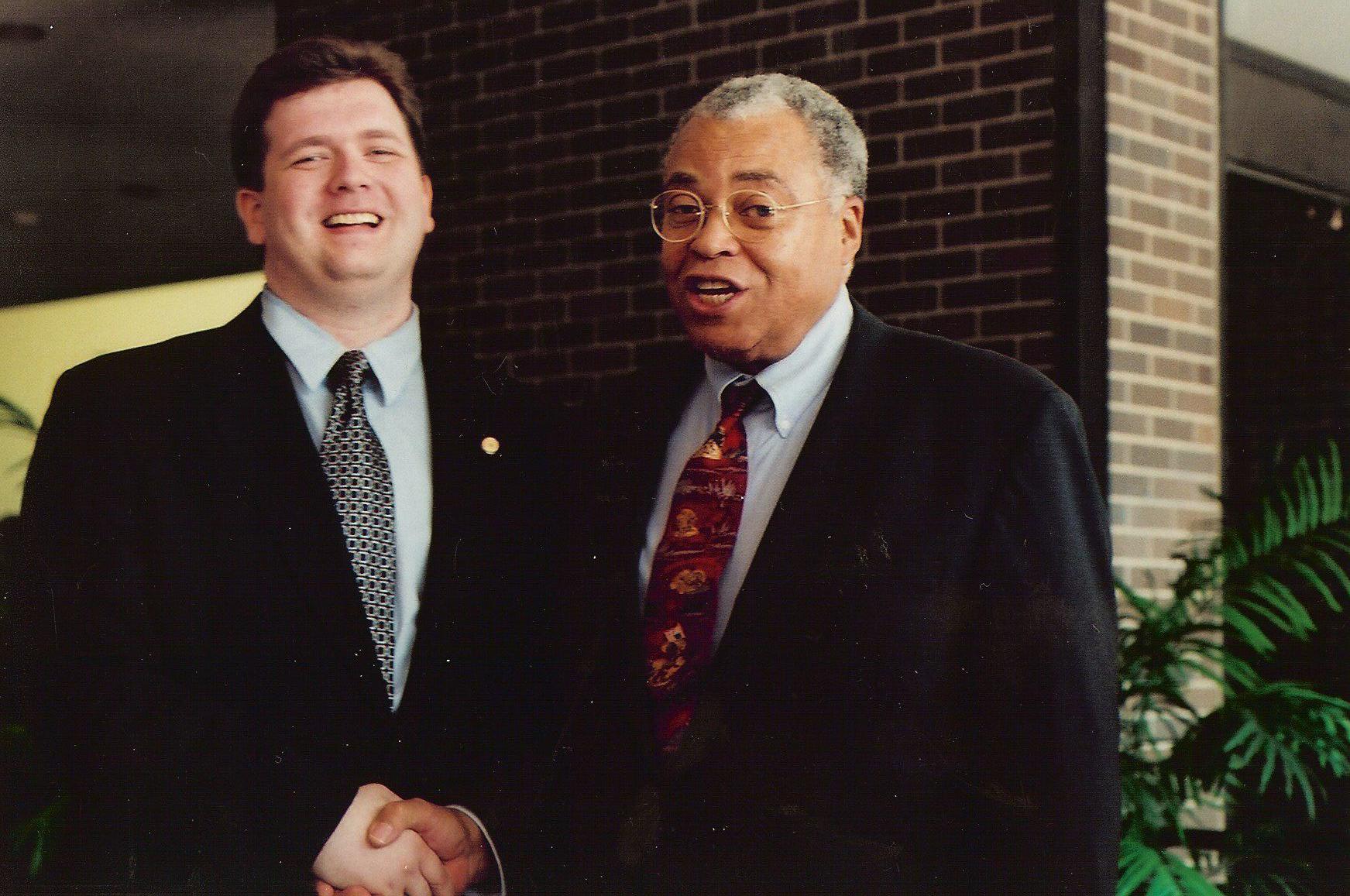In this detailed indoor image, two middle-aged men are warmly shaking hands while smiling and looking directly at the camera. The man on the left, identified as James Earl Jones, is adorned in a black tuxedo over a white collared dress shirt, accented by a red tie with a subtle printed design. He sports round glasses with gold frames and has short, graying hair. Jones appears to be in the midst of speaking, his mouth slightly open. The man on the right, who appears younger, is also clad in a black tuxedo paired with a white dress shirt and a black tie featuring a repeating square pattern. He has brown hair, lighter skin, and is adorned with a golden pin or badge on the right side of his tuxedo. Both men are under indoor lighting with a visible source of light in the top left. The setting features a brick wall that seemingly serves as a structural pillar, complemented by the large leaves of a plant on the right. The background also hints at possible doorways or hallways, enhancing the indoor ambiance.